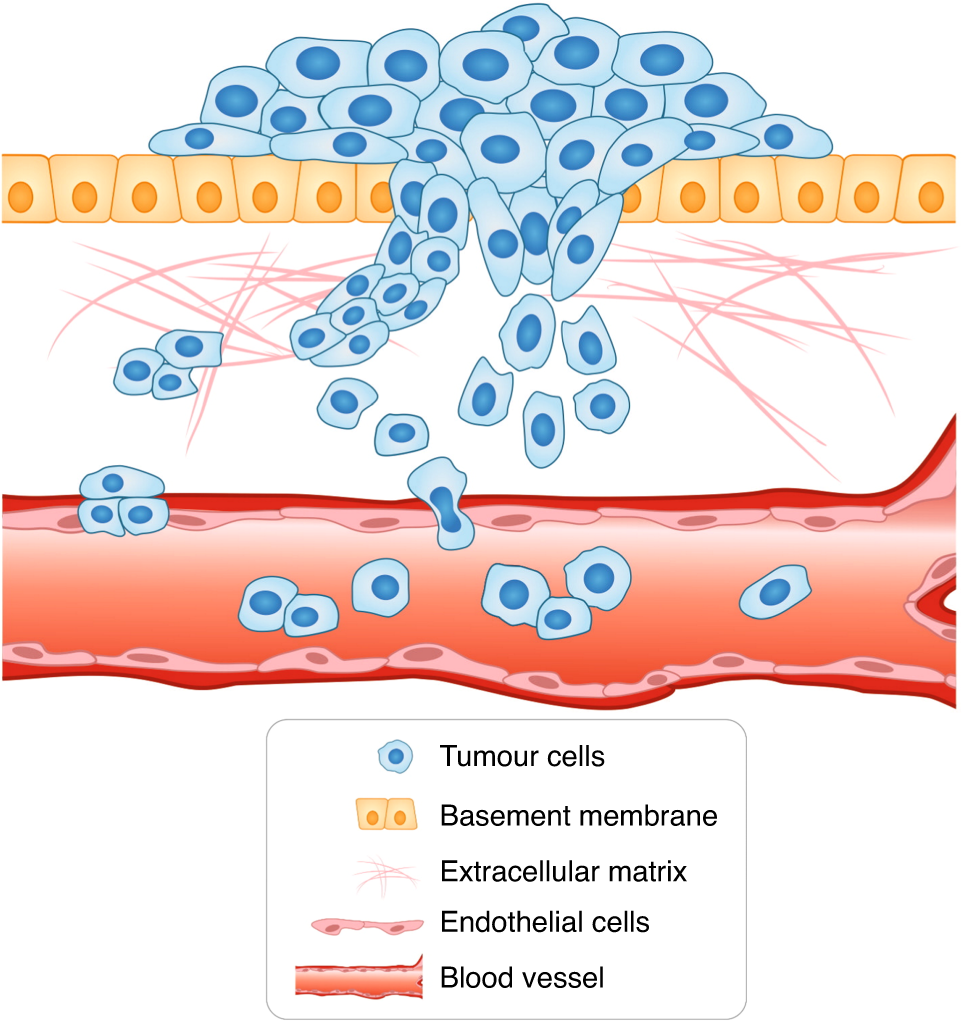The image appears to be a detailed, animated illustration from a scientific textbook, depicting various cellular structures and a blood vessel. At the bottom, there is a thick red tube labeled as a blood vessel, which transitions from dark red at the top and bottom sections to a more reddish hue in the center, with visible flow inside. Above this, there are endothelial cells represented by thin pink and red lines encasing the blood vessel. 

The extracellular matrix is depicted as a white area containing thin pink lines situated just above the endothelial cells. A straight layer of squares with yellow circles inside, identified as the basement membrane, sits on top of the extracellular matrix. Above this membrane, a row of blue cells, labeled as tumor cells, is piled up, resembling structures that almost look like fried eggs with blue centers.

The entire scene is set against a bright white background, enhanced by clear and precise lighting which makes the colors and structures distinctly visible. A small key or chart at the bottom of the image clearly labels each cell type: the blue sections as tumor cells, the yellow and orange squares as the basement membrane, the thin pink lines as the extracellular matrix, the pink and red areas as endothelial cells, and the thick red section as the blood vessel. This detailed depiction highlights the arrangement and relationship between these cellular components.